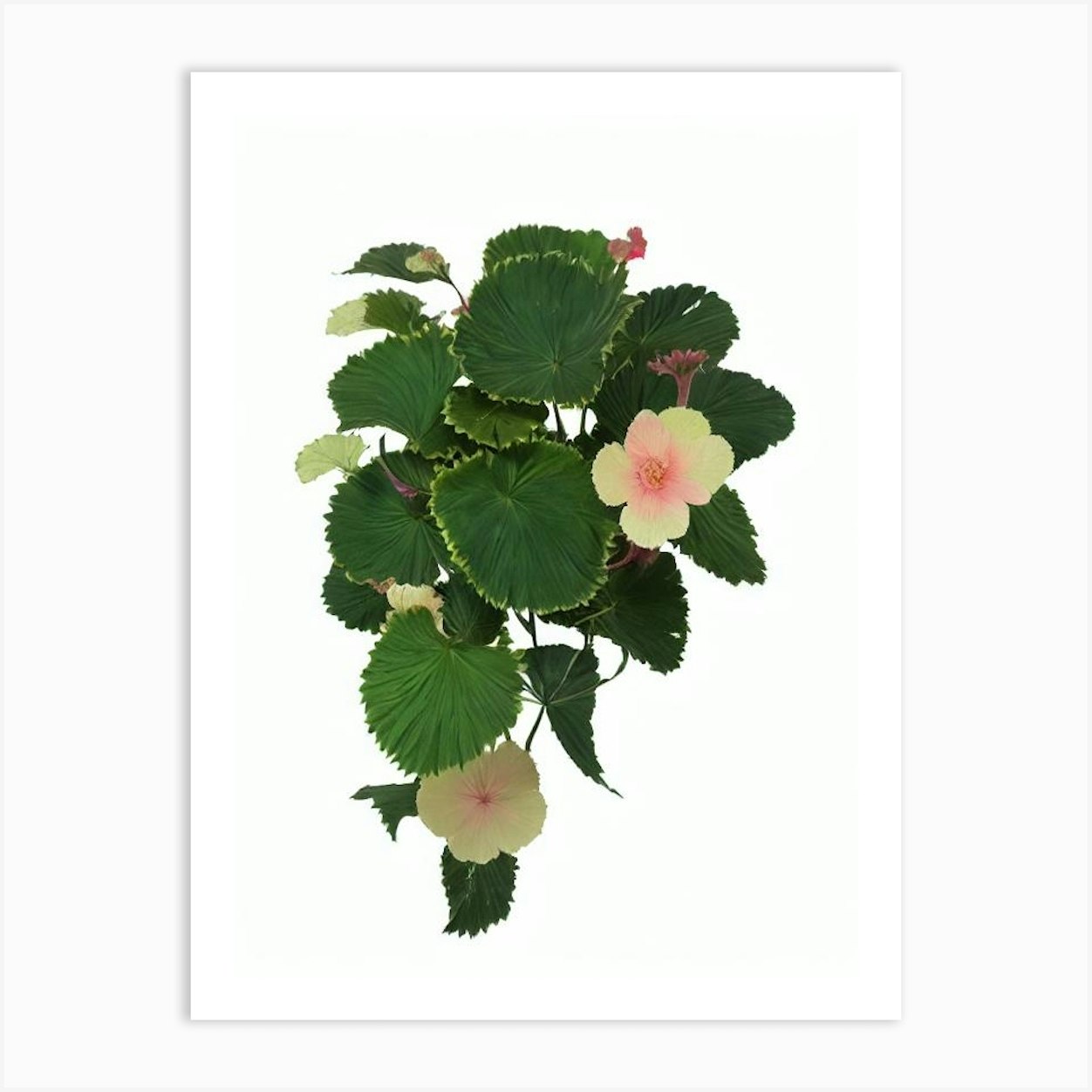The image is of a highly detailed, realistic painting of flowering plants, depicted on an 8x10 inch piece of paper with a slight drop shadow, emphasizing depth against a white background. The central feature is a cluster of predominantly dark green, round leaves with lighter edges, reminiscent of lily pads, arranged densely at the top and sparser toward the bottom. Among these lush leaves are various flowers and buds: cream-colored petals with pinkish centers, notably one circular flower at the bottom and another at the top right. Scattered throughout are unopened buds, some dark purple and some lighter pink. Notably, on the top center of the plant is a slightly open L-shaped petal or bud, colored in shades of pink or purple, adding an intriguing detail to the composition.